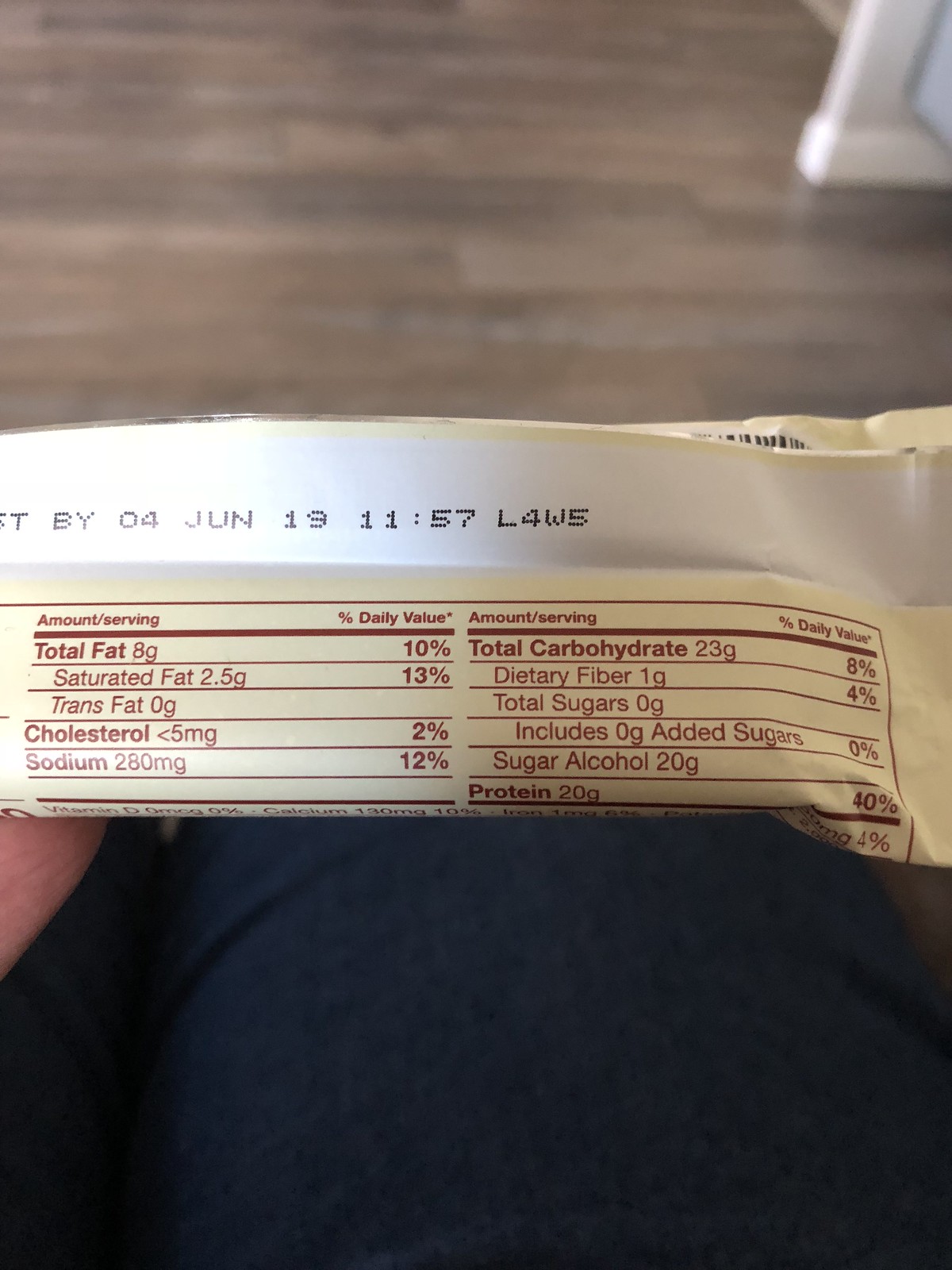The photograph captures a close-up of someone with a chubby gut, wearing a navy blue short-sleeved shirt, as they examine the nutritional facts on an eggshell-colored food wrapper adorned with burgundy font. The wrapper, partially folded, reveals nutritional details highlighted in black and red ink, specifying values such as 8 grams of total fat (10% DV), 2.5 grams of saturated fat (13% DV), 0 grams trans fat, 2% DV cholesterol, 280 milligrams of sodium (12% DV), 23 grams of total carbohydrates (8% DV), 1 gram of dietary fiber (4% DV), 0 grams of total and added sugars, 20 grams of sugar alcohol, and 20 grams of protein (40% DV). The expiration date on the food package reads June 4th, 19. The package is laid on the person's knee, clad in dark blue jeans. In the background, a blurred wooden floor and an indistinct white rectangular object, possibly a piece of furniture, are visible, emphasizing the detail on the wrapper.